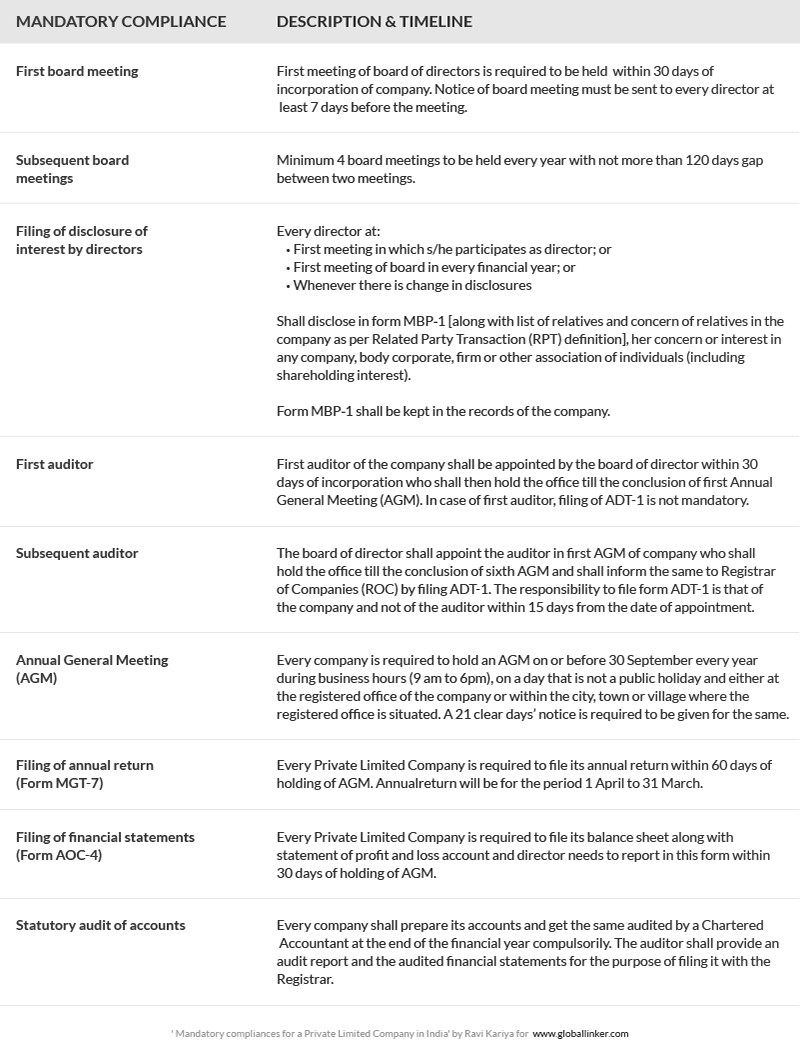**Detailed Caption:**

This is a screenshot of mandatory compliances for a private limited company in India, created by Ravi Kariya for www.globallinker.com. The top of the page features the headings "Mandatory Compliance," "Description," and "Timeline." The document details various compliance requirements:

1. **First Board Meeting**: It is mandatory for the first meeting of the board of directors to take place within 30 days of the company’s incorporation. A notice for this board meeting must be sent to every director at least seven days in advance.

2. **Subsequent Board Meetings**: A minimum of four board meetings must be held every year, with no more than a 120-day gap between any two meetings.

3. **Filing of Disclosure of Interest by Directors**: Every director is required to disclose their interest in Form MBP-1:
   - At the first meeting they participate in as a director.
   - At the first board meeting of each financial year.
   - Whenever there is a change in previously disclosed interests.
   
   This disclosure should include a list of the director's relatives, concerns, or interests in any company, body corporate, firm, or other association of individuals, in line with the Related Party Transaction (RPT) definition. The Form MBP-1 must be maintained in the company’s records.